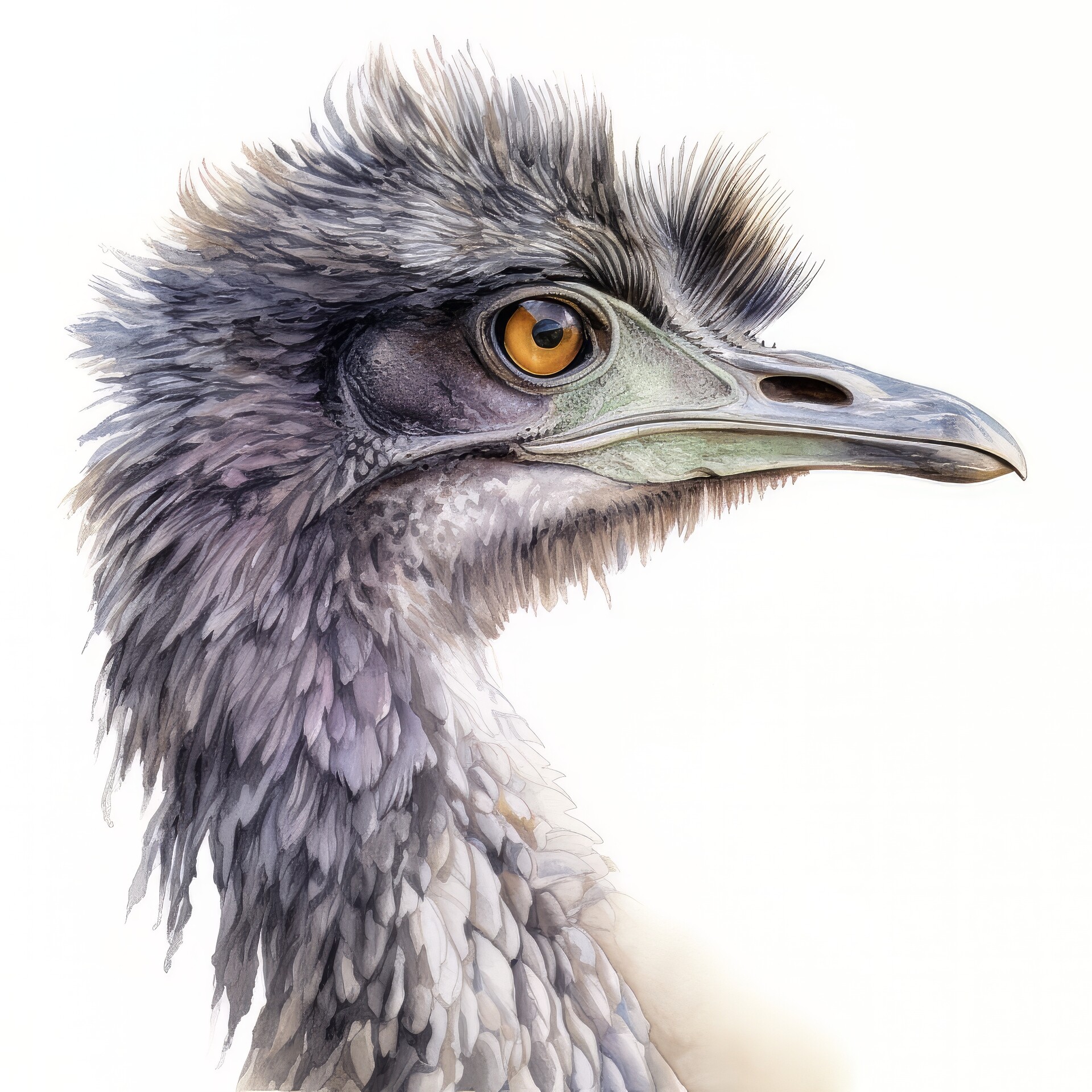The image is a detailed vertical illustration of a bird's head, possibly an ostrich or an emu. The bird is shown from the neck up, in a side profile, looking to the right with the beak pointing in that direction. The background is plain white, emphasizing the bird's features. The bird's large, striking eyes are a notable brown or gold color, set within a featherless region around the eye which adds to their prominence. The bird has a long, powerful gray beak that extends both under the chin and up to the eye, with a noticeable nostril hole on the side. The feathers along the neck are thick and become progressively more feathery and wild as they reach the top of the head, sticking out in various directions. The coloration of the feathers is predominantly gray, with variations that include lighter and darker shades, as well as hints of black and white. The bird's appearance combines solid and delicate details, with the feathers around the head and neck looking plush yet slightly disheveled.